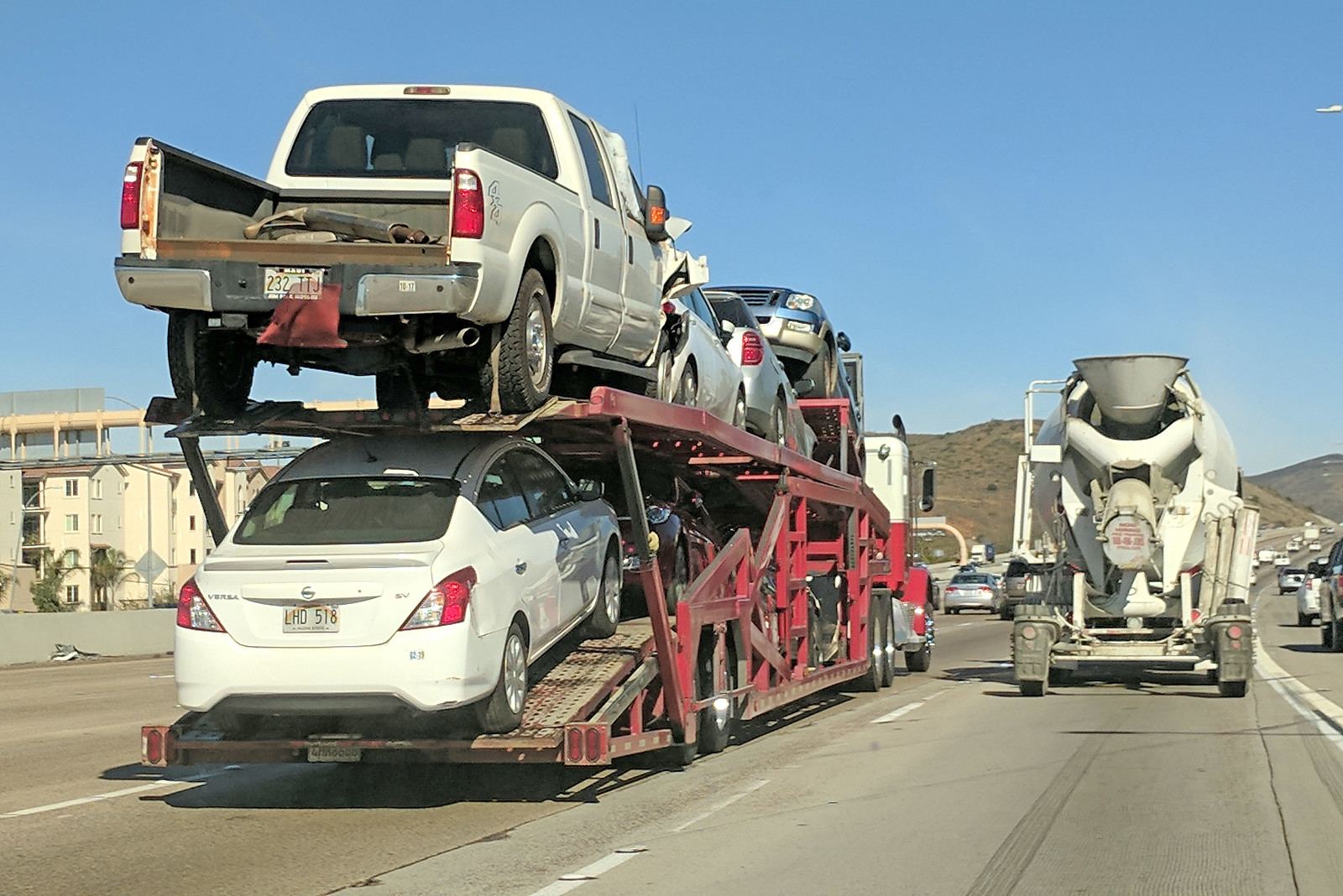In this vibrant daytime photograph taken from the perspective of a car driving on a sunny highway in the United States, a detailed scene unfolds. The primary focus is on two vehicles—a massive cement mixer and a car transporter truck—moving in front of the observer’s vehicle. The cement mixer, sporting a distinctive red writing on its covered spout, is located in the rightmost lane. Meanwhile, the car transporter truck, positioned one lane to the left, features a striking design with a white upper cab and a red lower section, along with a black smoke pipe.

This transporter is towing an impressive array of vehicles, divided between two levels. On the lower level, towards the rear, a white Nissan Versa with a license plate "LHD 581" and a rainbow decal can be seen. In front of it, there's a red or maroon car, followed by several more vehicles. On the top level, the striking feature is a white pickup truck missing its rear door, which also has a license plate "232 TTJ" partially obscured by a mysterious red or transparent image. The flatbed of this pickup carries what might be a piece of tailpipe or exhaust, adding to the chaotic, almost surreal assembly of this vehicle transport scene. Additionally, other cars, including a potentially damaged one, a white SUV, and a blue SUV, are precariously stacked on this upper level. 

In the surrounding scenery, the left side of the image reveals tall, white apartment buildings, standing out against the backdrop of brown, dry hills. These structures provide a sense of location and contribute to the bustling, multifaceted atmosphere of the freeway. The highway lanes are marked with long white lines and round bumpers, indicating a well-traveled road under the glare of the sun, truly capturing a moment of dynamic motion and complexity on an American road during daylight.